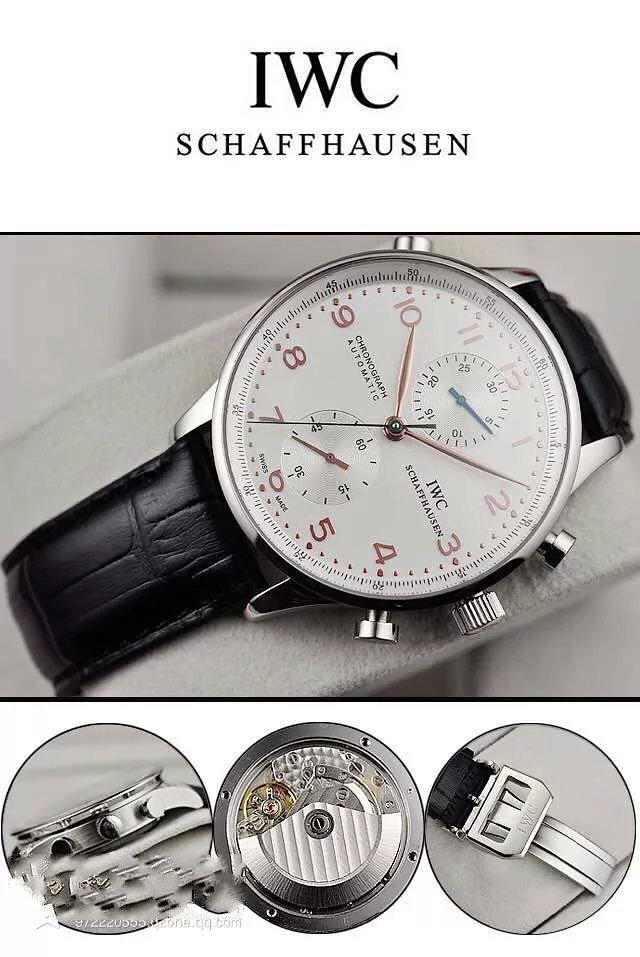This advertisement showcases the luxurious IWC Schaffhausen watch, renowned for its Swiss craftsmanship. The layout features a triptych montage, with the central image prominently displaying the watch on a sleek, gray jewelry box. The primary focus is on the elegant watch face, accented with striking red numerals and indices. The detailed close-up highlights the meticulously designed black leather strap and reveals the intricate features of the watch's face. Notable elements include the second hand, a date indicator, and sub-dials that likely serve additional functions. The watch is identified as a chronograph, emphasizing its automatic movement and precision. Three adjustment knobs are visible, which are used to set the date, time, and other functionalities. The bottom section of the advertisement provides finer details, further illustrating the watch’s specifications and luxurious appeal.